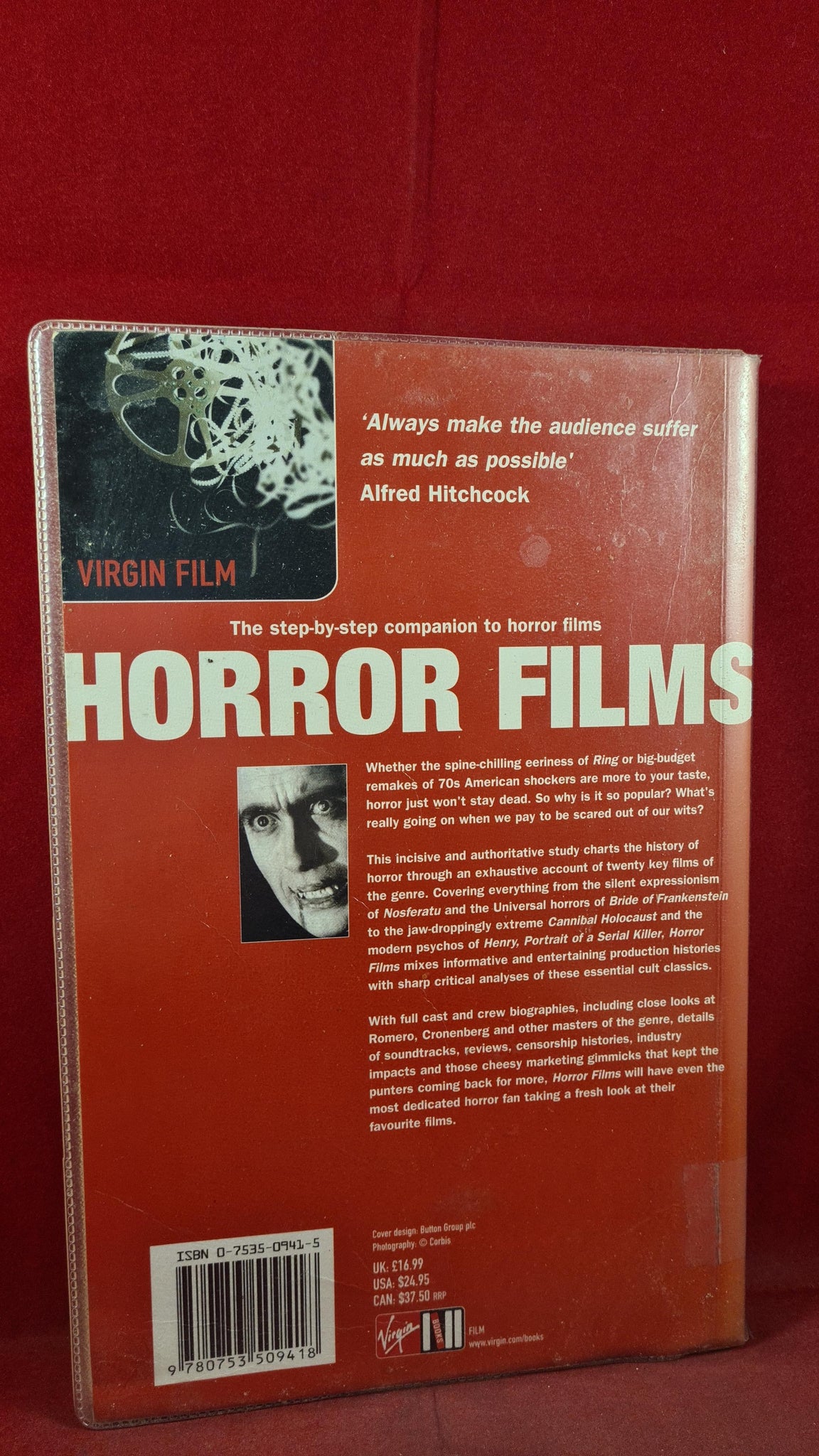This image captures the back cover of a DVD case propped against a red-painted brick wall. The dominant color of the case's backside is a deep red, showcasing various elements in black, white, and red. In the upper left corner, there's a black and white image of a film reel with red text that reads, "Virgin Film," alongside an Alfred Hitchcock quote: "Always make the audience suffer as much as possible." The central part of the cover features a large title, "Horror Films," beneath which lies most of the descriptive text. A haunting black and white photo of a man with a drop of blood at the corner of his mouth, evoking a vampire-like appearance, adds to the eerie atmosphere. The text also mentions this being a "step-by-step companion to horror films." Additionally, a barcode is visible in the bottom left corner.